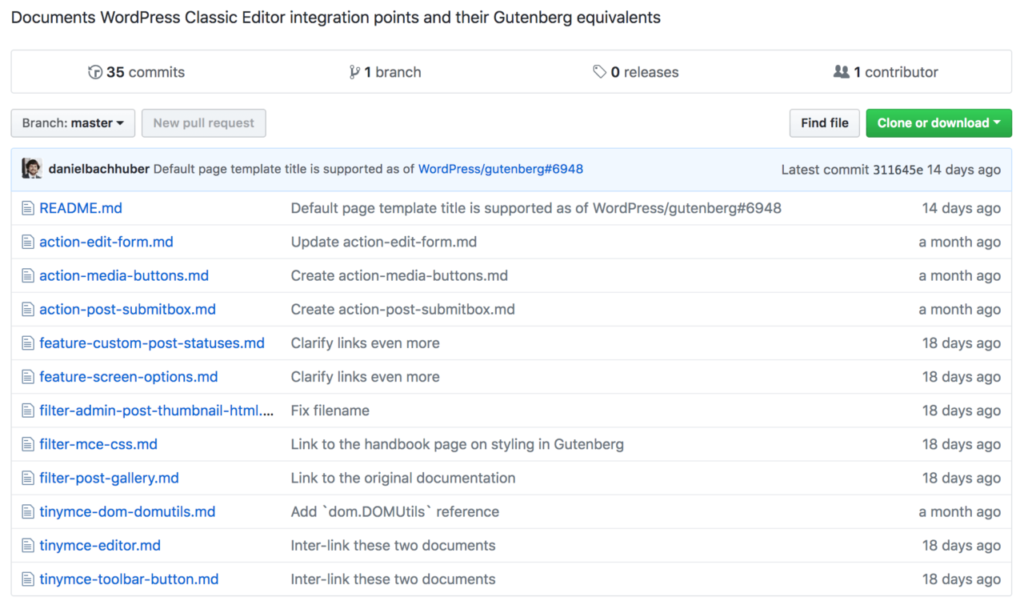This screenshot captures an image of a web or application development platform, likely GitHub or a similar platform like WordPress, utilized for developing websites or applications. At the top center, there is a prominent title in large black text reading "Documents: WordPress Classic Editor Integration Points and Their Gutenberg Equivalents," indicating the subject of the project. 

Directly below this title is a horizontal white box with a light gray outline containing vital project statistics: "35 commits," "1 branch," "0 releases," and "1 contributor." These terms pertain to the software development lifecycle, where "commits" refer to individual changes or updates made to the project, and "branch" refers to a separate working version of the project.

The main section of the image is predominantly filled with rows listing different files or changes within the project. The file names, written in blue text, include titles like `readme.md`, `action-media-buttons.md`, and `filter-post-gallery.md`. The "md" file extension suggests these are Markdown files.

In the center of each row, descriptions in gray text summarize recent changes made to the respective files, with comments such as "clarify links even more" and "fix file name." These descriptions provide context for the updates or modifications. On the far right of each row, another set of gray text indicates the last update timestamp for each file, displaying information like "14 days ago" or "a month ago."